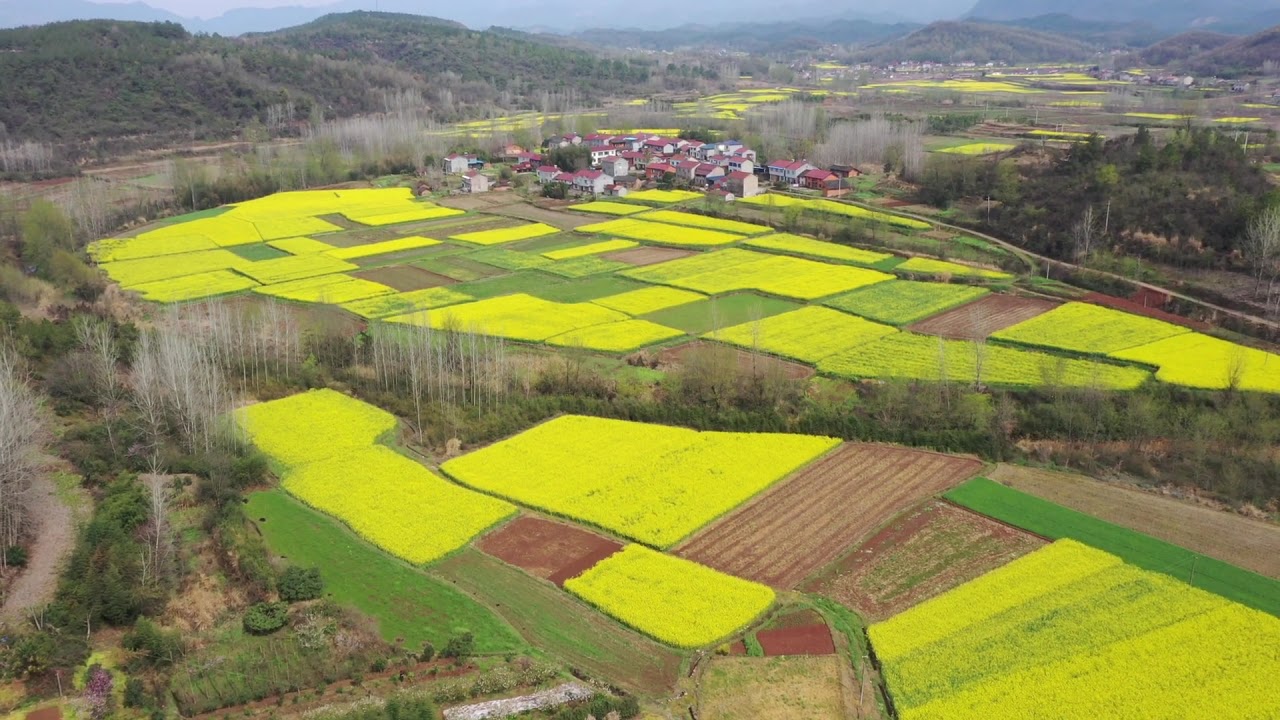This overhead photograph captures a small town nestled amidst extensive farmland, taken from a high elevation. In the center, there is a clustered residential area where numerous houses are closely situated together, suggesting a tight-knit community or possible agricultural processing buildings. Surrounding the town are various rectangular plots of farmland, distinctively divided into sections. The fields exhibit varying stages of cultivation: some are lush green, indicating flourishing crops, while others are a vibrant yellow, possibly fields of flowering plants. A few plots remain bare and brown, awaiting planting. On the periphery of the farmland, rolling hills covered with dense trees and bushes frame the scene. In the distance, the horizon stretches out to faint, tree-covered mountains under a partially overcast sky, adding depth and a sense of vastness to the picturesque rural landscape.